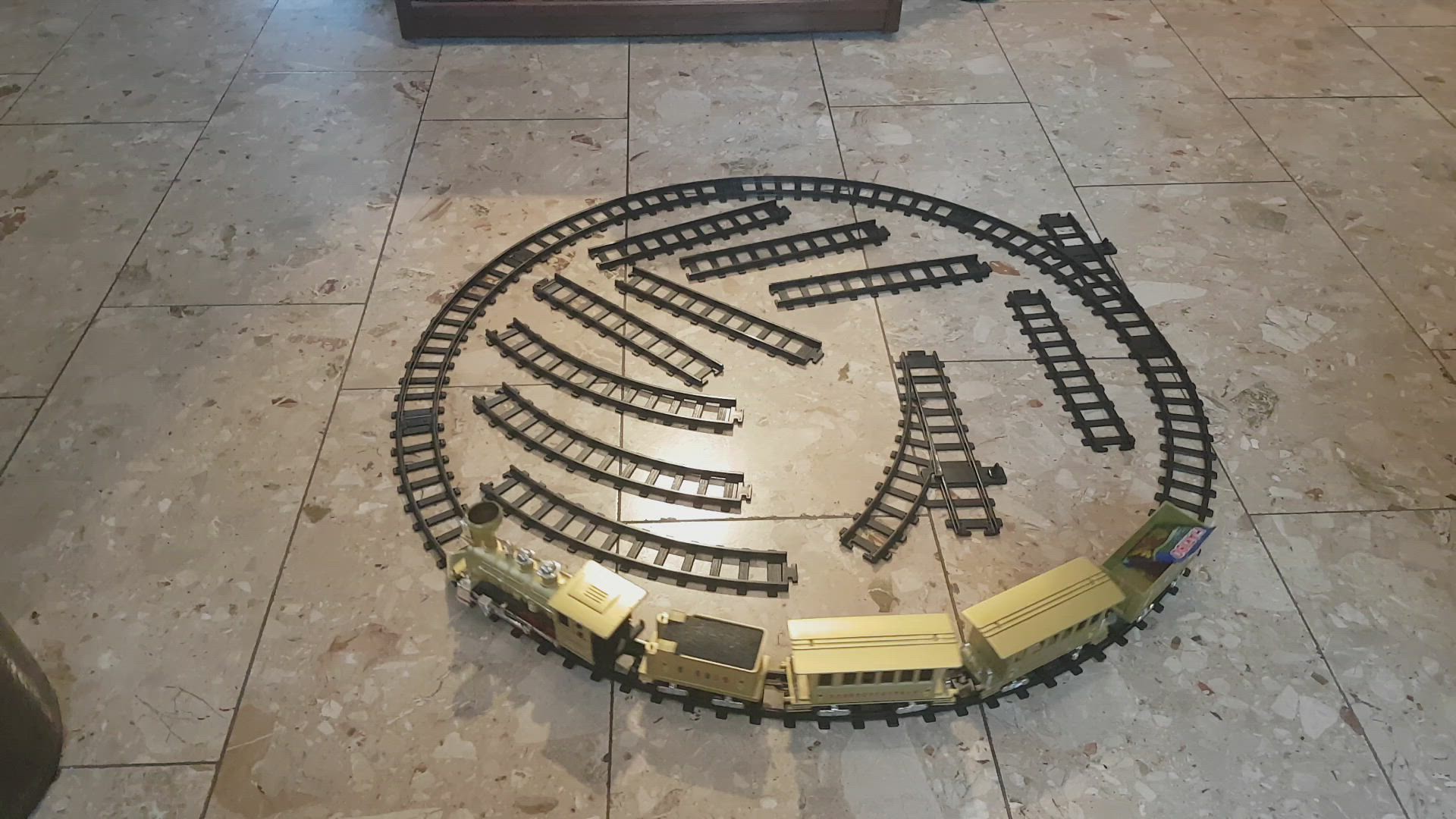The photograph depicts a detailed zoomed-in view of a golden model train set arranged in a circular formation on a beige-tiled floor. The tiles have a marble-like appearance with specks of white, darker beige, and brown. The train set includes a main engine, three cars, and a caboose, all positioned on black tracks. Inside the circle of tracks, there are various spare pieces. Notably, the last car is open-topped, containing a blue packet of Haribo gummy bears, placed under a light source.